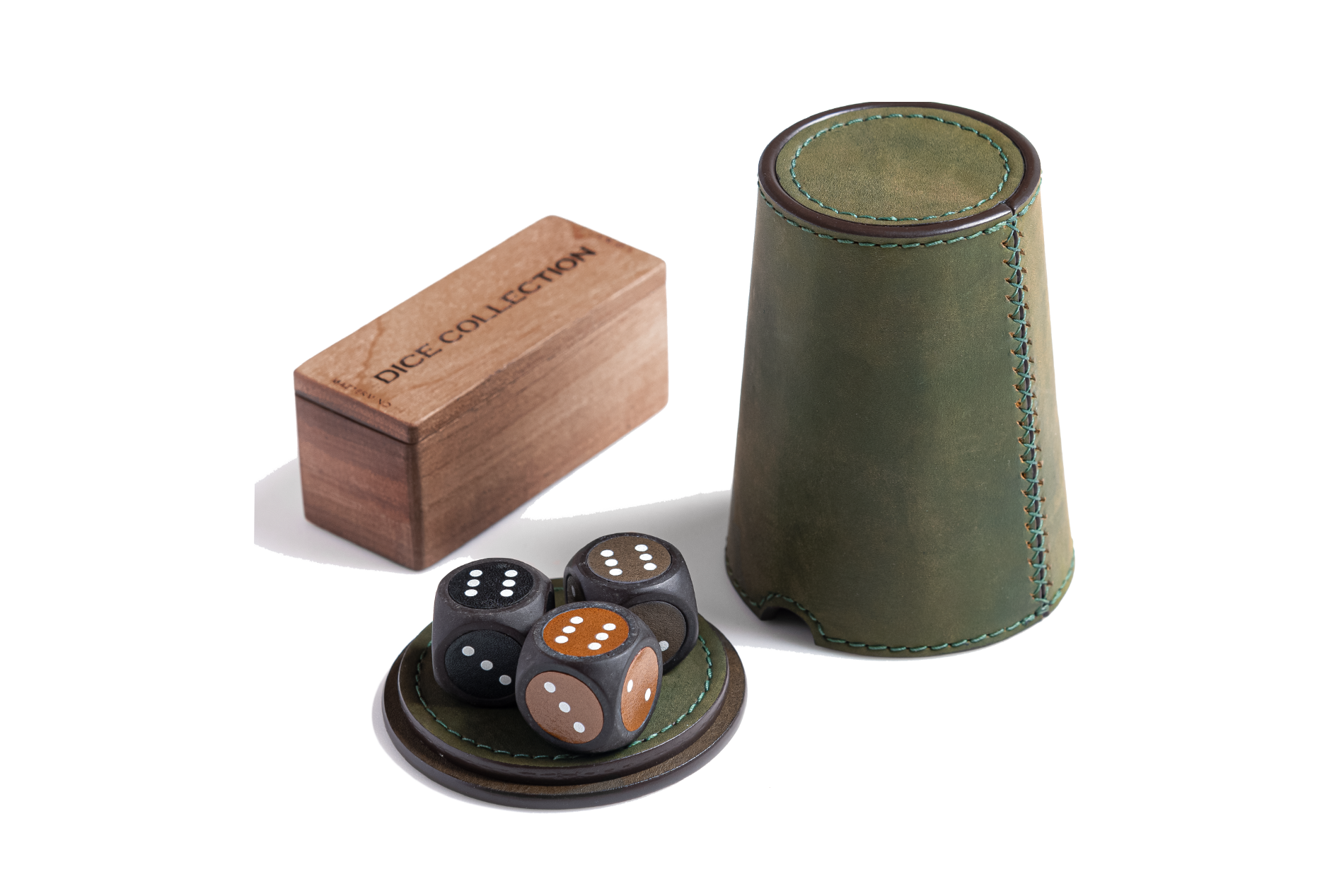Against a stark white background, a meticulously arranged game set sits, bathed in light from the three o'clock position, casting shadows toward nine o'clock. Central to the image is an olive green leather coaster with precise white stitching, bordered by a dark brown rim. Atop this circular base are three black dice, each displaying a six on the top face. The dice feature diverse color palettes on their sides, incorporating dark hues like brown and red. 

In the upper left corner of the scene, a light brown wooden box labeled "dice collection" is positioned diagonally, tilting upward toward the one o'clock direction. This rectangular box has a removable thin top. Meanwhile, in the upper right corner, an olive green leather cup—similar in design to the coaster with matching stitching and brown rim—lies turned upside down, its cylindrical shape reminiscent of a thimble.

Together, these objects form an evocative tableau of a game in readiness, each item meticulously placed to highlight their textures and colors against the pristine background.